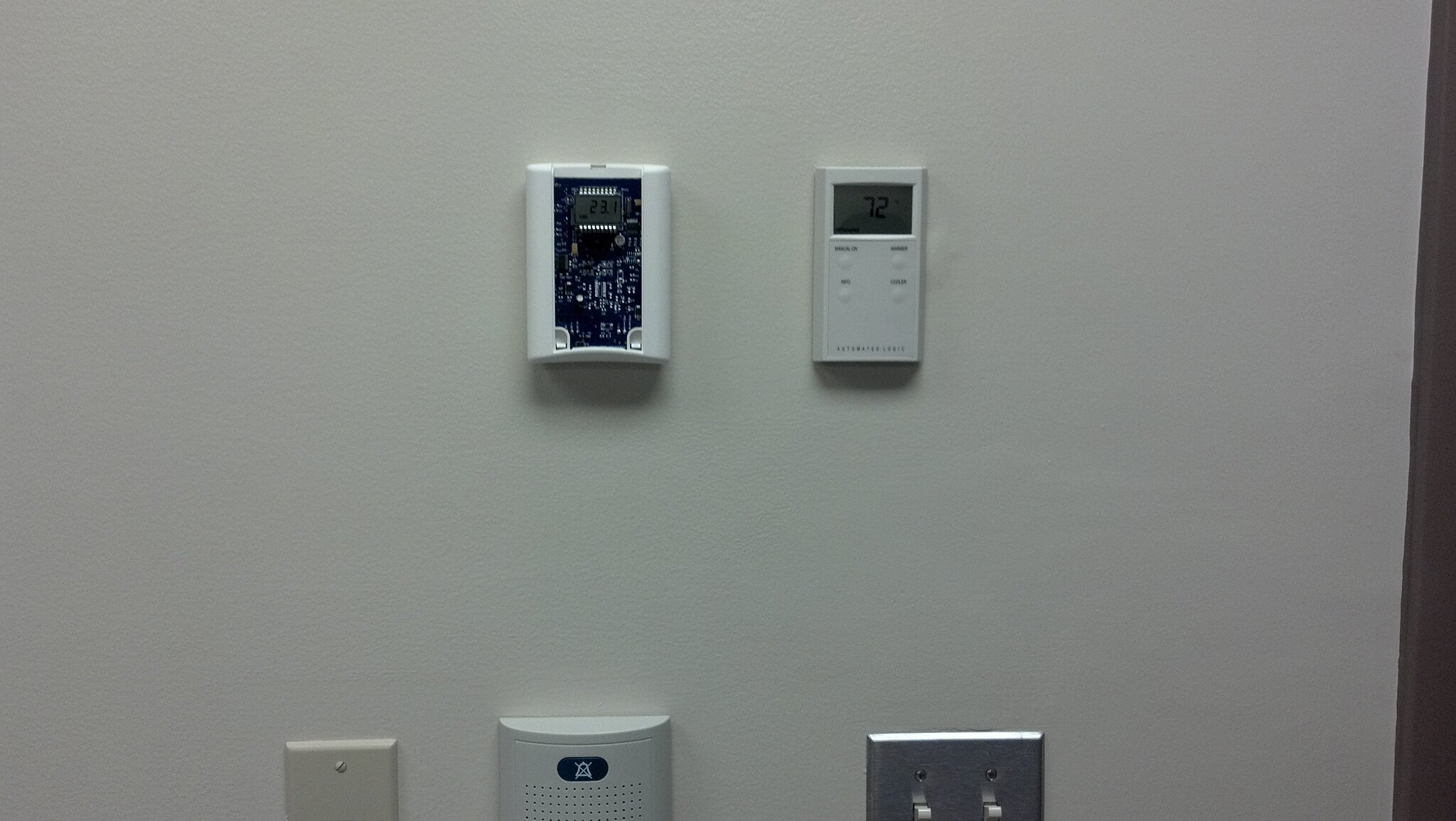This photograph captures a detailed view of a light gray wall densely populated with various electronic devices. On the left side of the wall, an HVAC thermostat with its cover removed reveals intricate electronics. To its right, a controller, possibly for a furnace or air conditioner, features a clearly readable LCD screen displaying the temperature as 72°F. The exact type of unit controlled remains indeterminate, as the controller could belong to either a central air conditioning system or a split-type unit. In the lower right corner, a silver two-gang outlet plate with two switches is visible. The center bottom of the image showcases a motion detector, likely serving as an intruder sensor. The lower left area displays a blank mounting plate covering some wiring. Additionally, the far right edge of the image reveals the dark walnut molding of a doorway, offering a touch of contrast to the otherwise utilitarian scene.